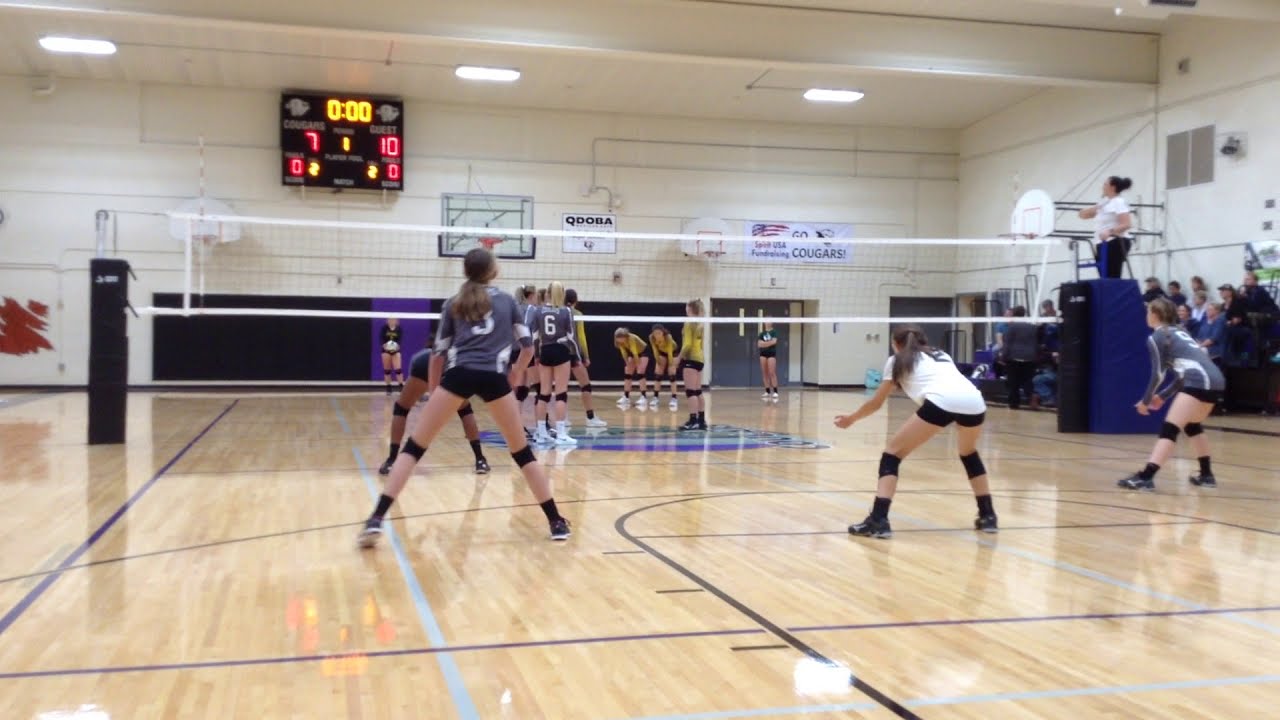The image captures an indoor girls' volleyball game in progress within a gymnasium, viewed in landscape orientation from across the gym floor. On the near side of the net, several players with gray jerseys and black shorts are facing away from the viewer, each wearing black knee pads and black or white sneakers. One player stands out in a white jersey. On the far side of the net, other players, some in blue and white shirts, are bending down and ready to play. A few individuals in yellow shirts can be seen in the background. The volleyball net is predominantly white.

A digital scoreboard in the distance shows no time left, with the home team, labeled 'Cougars', scoring 7 points while the Guests have 10 points, both scores illuminated in red lights. The scoreboard hangs above a far wall adorned with a mounted basketball hoop and various signs, including one white sign with a partial American flag and the words "Go Cougars!" in dark blue.

Positioned on the right side of the image is a blue podium with a female referee standing on top, wearing a white shirt, dark trousers, and dark hair tied back. Spectators are seated in bleachers, observing the game attentively. The scene is a realistic and dynamic portrayal of a high school volleyball match, with attention to the action on the court and the surrounding environment.